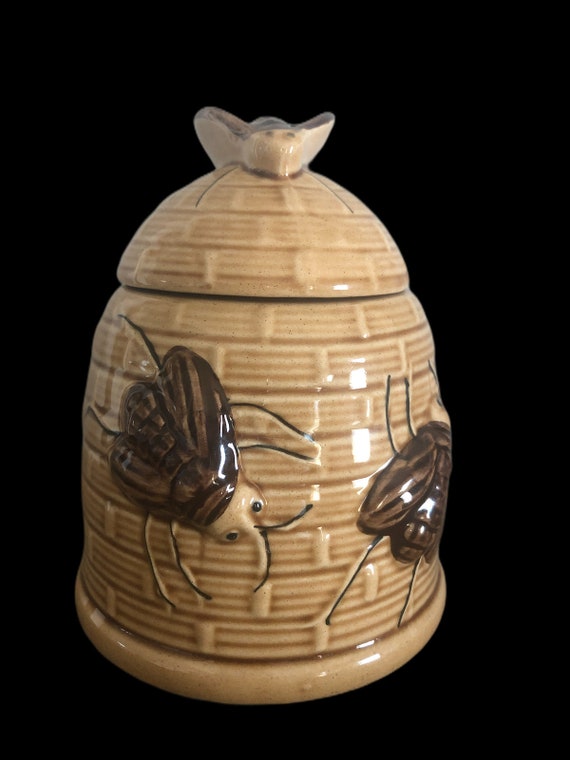The image showcases a small, tan-colored clay pot with a lid, resembling a cookie jar, possibly designed for storing honey given its features. The pot features a detailed, glazed finish with a golden brown hue and a pattern resembling brickwork or a beehive. Superimposed on this pattern are two brown and light brown creatures, likely meant to be bees or similar insects, characterized by black legs, honey-colored heads, long skinny legs, and pointed snouts with visible eyes. The jar sits against a completely black background, emphasizing its intricate details and rendering the scale somewhat unclear, though it appears to be the size of a small salt shaker. The lid of the jar includes a small handle, possibly designed to resemble another small animal, adding to the whimsical and detailed nature of the piece.